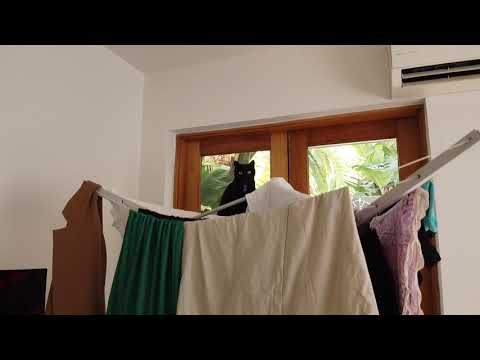The image captures a serene indoor scene featuring a black cat as the focal point. The cat, with its piercing green eyes and erect ears, sits calmly in front of a window framed by light-colored wood. Through the window, a lush, sunlit expanse of greenery is visible. Below the window, an indoor drying rack is prominently occupied with various pieces of fabric - brown, green, beige, and pink. The surrounding environment is clean and modern, with white-painted walls and ceiling. An air-conditioning unit with open grills is mounted on the top right corner of the room, hinting at a comfortable, climate-controlled space. The cat, poised and still, gazes directly into the camera, providing a juxtaposition of calm amidst the practical, everyday setting of drying laundry.